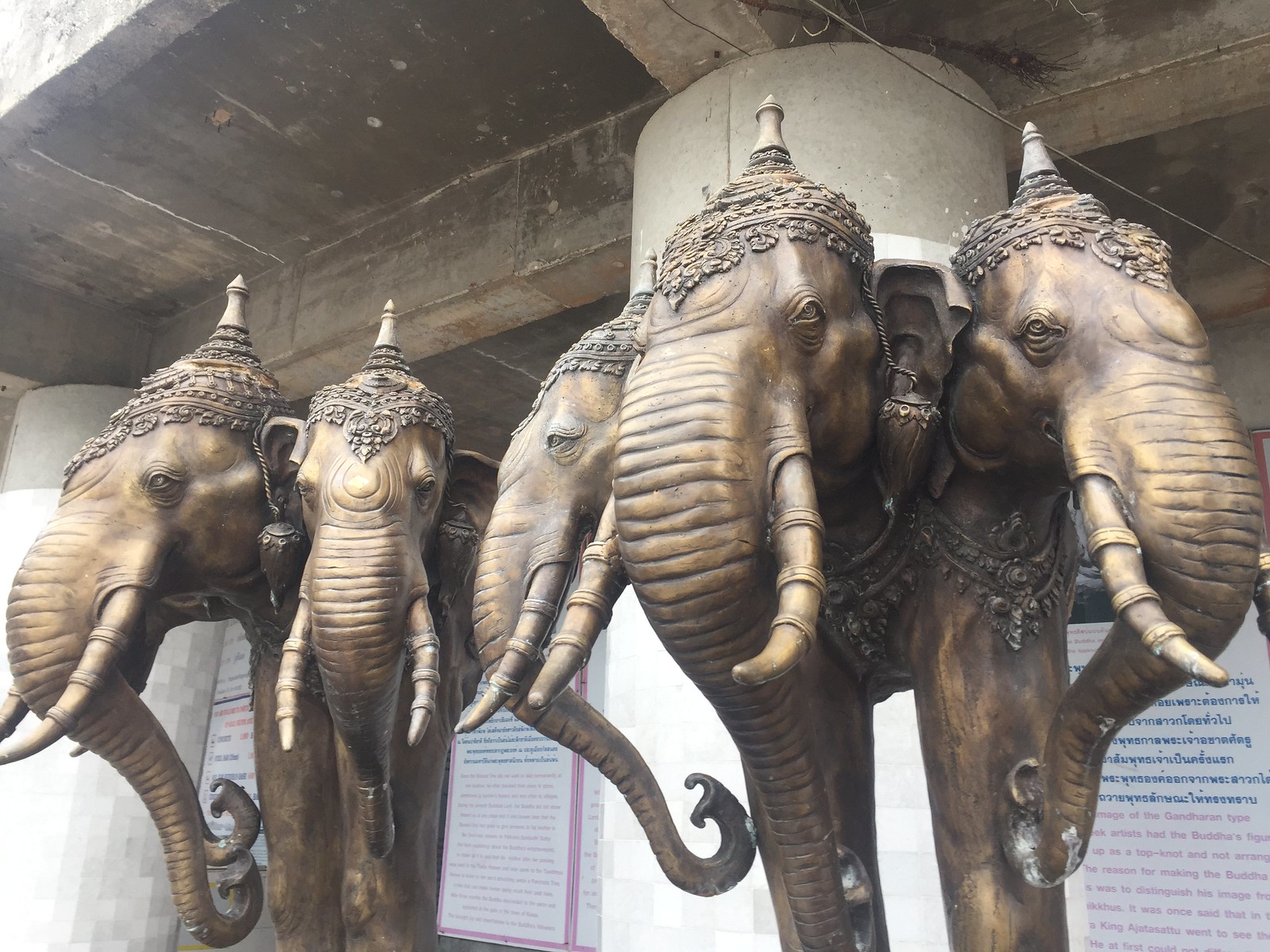This image depicts a series of intricately detailed bronze statues of elephants, which serve as ornate columns supporting a stone platform, possibly in a historical or cultural display. Each column consists of three elephants, adorned with elaborate headdresses, necklaces, jewelry, and large tusks. The elephants' trunks are artistically curled towards their bodies, with one elephant posing with its knee raised as if in motion. Behind these statues, there is a white wall featuring inscriptions in an unfamiliar language, with blue writing on top and red writing below. The scene is framed by concrete support beams above, enhancing the grandeur and significance of the artistic installation.